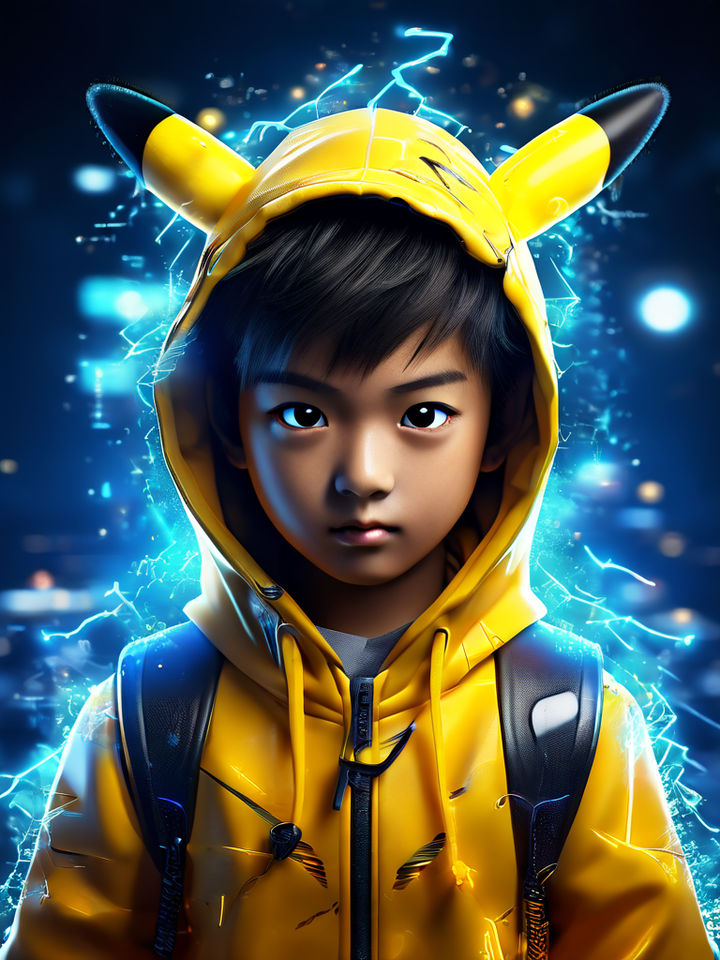This is a highly detailed, computer-generated image of a young boy, possibly Asian, around the age of 10. He has light brown, coffee-colored skin and black hair swept across his forehead to the left. His facial expression is quite serious. The boy is wearing an oversized yellow hoodie styled after Pikachu, complete with cylindrical ears that have black tips. Over his shoulders, you can see the substantial black leather straps of a backpack. The scene is electrified with a turquoise blue and white light, making it appear as though he is generating or emanating electricity. The background is blurred with blue lights and a darker backdrop, further accentuating the boy as the central figure.